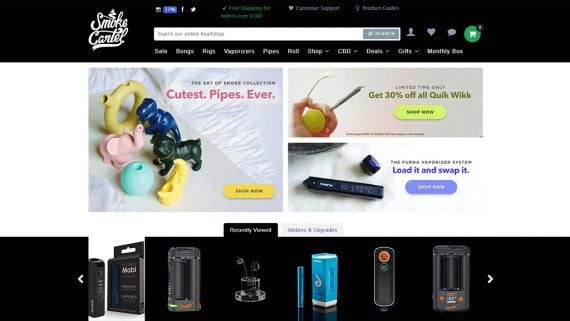A screenshot from the Smoke Cartel website, cropped to display only the browser window. At the top is a black rectangular header featuring a white "Smoke Cartel" logo in the upper left-hand corner. Despite the low image quality making some text hard to read, the top black-grey section includes navigational menus with buttons for browsing. There’s also a search bar, icons for user profile, favorited items, a speech bubble—presumably for help or support—and a green shopping cart icon.

The middle section of the screenshot showcases three clickable graphics, each hyperlinking to different sections of the shop. The first graphic highlights a selection of smoking pipes. The second promotes a "limited time only" 30% off sale. The third directs users to a "Load It and Swap It" vaporizer system section.

At the bottom is another black rectangular area featuring a carousel-style display of various products available for sale, allowing users to scroll through different items.